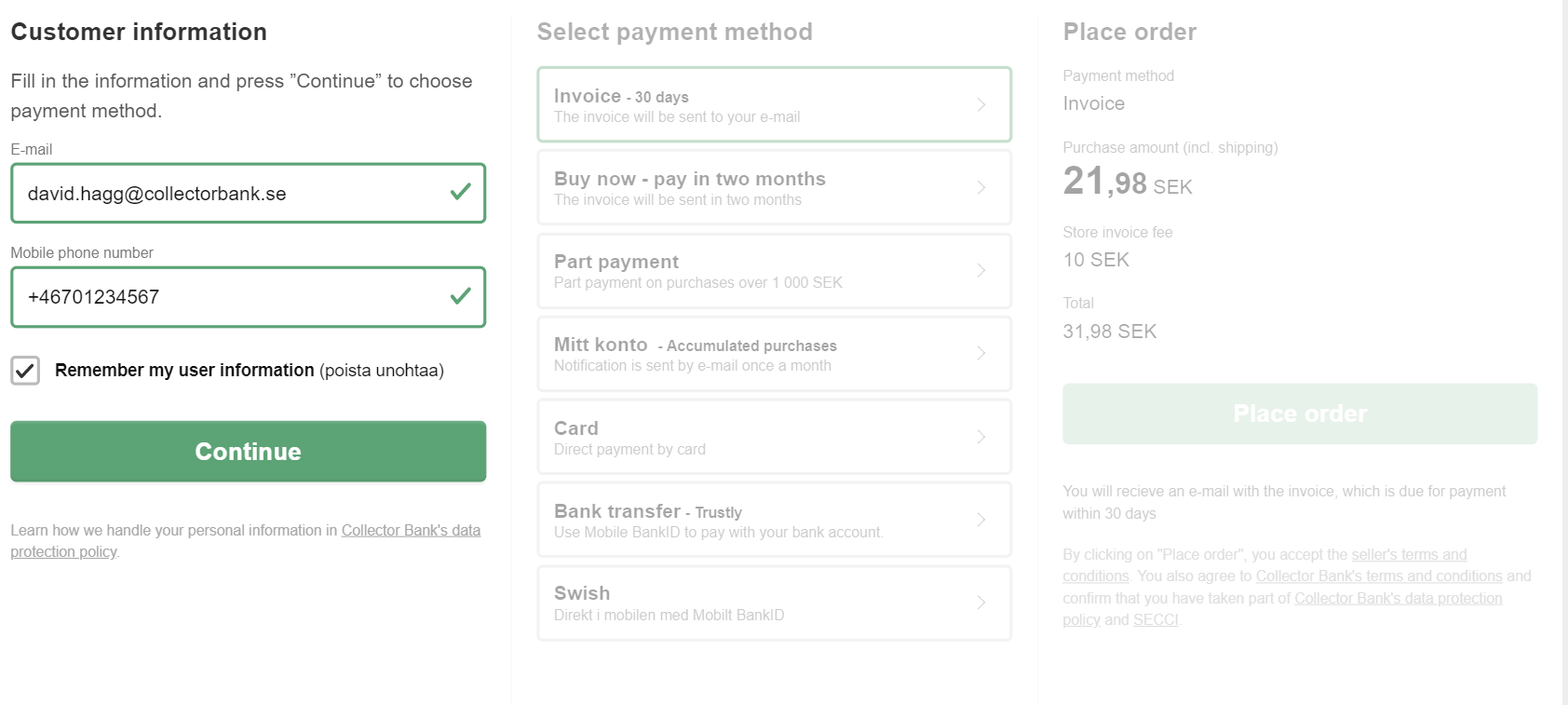In this image, we observe three aligned sections, each representing a step in the online checkout process. The first section on the left, which is highlighted, focuses on the customer's information. At the top, there's an instruction to fill in the customer details and press "Continue" to select a payment method. 

Within a green-bordered box, there is a field for entering the email address, followed by another green-bordered field for the phone number, specifically a mobile phone number. Additionally, an option to "Remember my user information" is checked, and below this, there is a "Continue" button.

The middle section, though not highlighted, pertains to the selection of the payment method. The available options include:

- **Invoice 30 days:** Payment is due 30 days after the invoice is issued.
- **Buy now, pay in two months:** The invoice will be sent in two months.
- **Part payment:** Accumulated purchases with a notification sent via email once a month.
- **Card:** Direct payment by card.
- **Bank transfer:** Using "Trustly," enabling payment with a mobile bank ID.
- **Swish:** Another mobile payment option.

Finally, the section on the right, also not highlighted, summarizes the order details and finalizes the purchase. It lists:

- **Place Order:** The button to complete the purchase.
- **Payment Method:** Currently selected as "Invoice."
- **Purchase Amount including Shipping:** 21,98 SEK.
- **Store Invoice Fee:** 10 SEK.
- **Total:** 31,98 SEK.
- **Place Order:** Button to confirm and place the order.

This detailed breakdown provides a comprehensive view of the checkout interface, guiding the user through the customer information input, payment method selection, and final order confirmation.